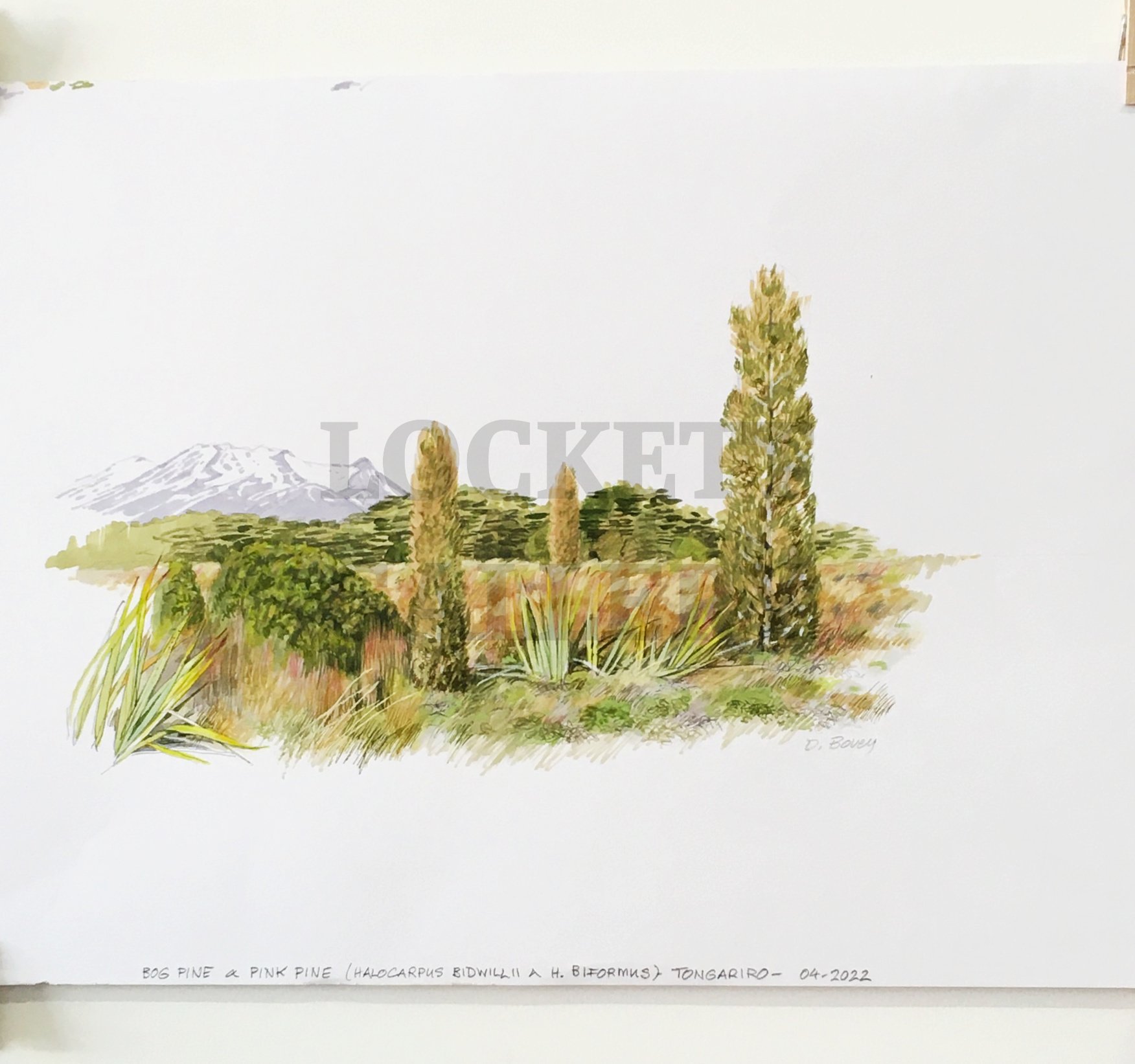This image features a light gray card set against a white background, showcasing a delicate illustration at its center. The drawing portrays a grassy area abundant with various types of vegetation, including green and brown grass, tropical plants, and shrubs. On the left, a short cactus is depicted, and to its right stands a taller, tree-like structure, probably a type of pine. The vegetation in the foreground includes aloe-like plants and other weedy flora. In the distance, a series of mountains or hills fades into the background, rendered in a watercolor style that blends seamlessly with the lightly colored card. 

The artwork, occupying just the middle portion of the card, appears as though it has been meticulously scanned. Behind the illustrated scene, the word "LOCKETT" is prominently printed in capital letters, potentially as an overlay. At the bottom of the card, small black text reads, "bog pine and pink pine. Hallocarpus bidwill A.H. biformis," with further notation "Tongariro 04-2022" indicating the date and location. The artist's signature is subtly placed in the very right-hand corner.